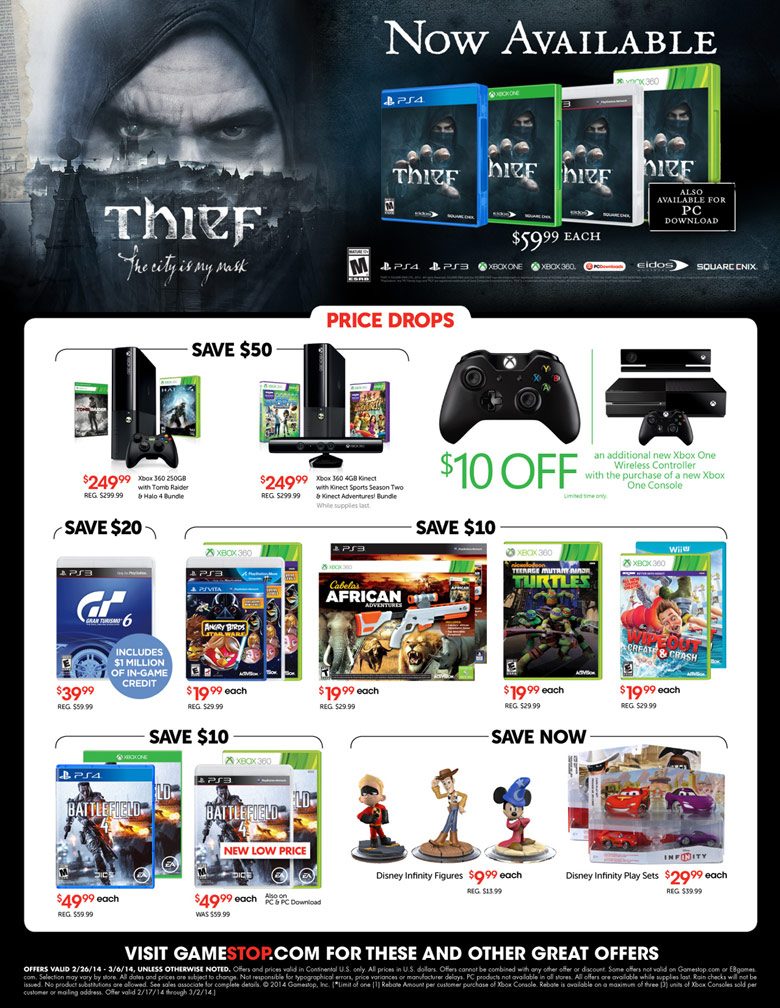The image showcases a promotional display for PlayStation 4 games, consoles, and controllers. The upper section features the game "Thief." On the left side of the top portion, there is a close-up image of the game's main character, a man clad in a hood with a mask covering his nose and mouth, revealing only his eyes and forehead. The background of the image is semi-transparent, presenting a dark, ominous landscape.

To the right of the character image, the text "Now Available" is prominently displayed. Additionally, an array of platform icons is visible, indicating that the game is available on multiple systems including PS4, Xbox One, Xbox 360, and PC. Below this, the price of the game is listed as "$59.99 each."

Directly beneath the main promotional area, there are several rows of PlayStation 4-related items arranged side-by-side, accompanied by detailed descriptions and pricing information.